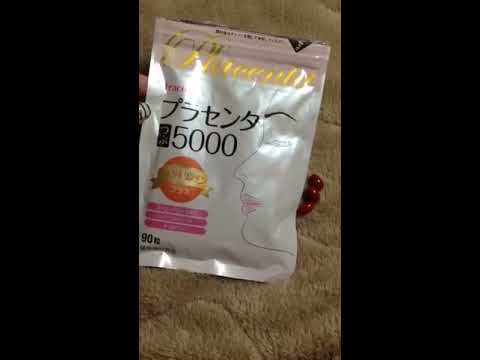The image features a package of what appears to be a Korean beauty or health product strategically placed on a textured surface, likely a blanket or carpet, with some decorative elements like beads scattered around. The package is centrally positioned and has been opened, revealing three red capsules laid nearby on the blanket. The package itself is primarily white with pink designs, adorned with yellow and black lettering, and contains a detailed caricature of a woman's face with her eyes closed. The text on the packaging is mostly in an Asian language, but the number "5000" is prominently displayed, indicating the quantity or strength of the contents. The ingredients and usage details are also visible on the package. A person with acrylic nails decorated in a black and white striped design is holding the bag in place for the photo. The image is bordered by black vertical bars on either side and measures approximately five inches by five inches.